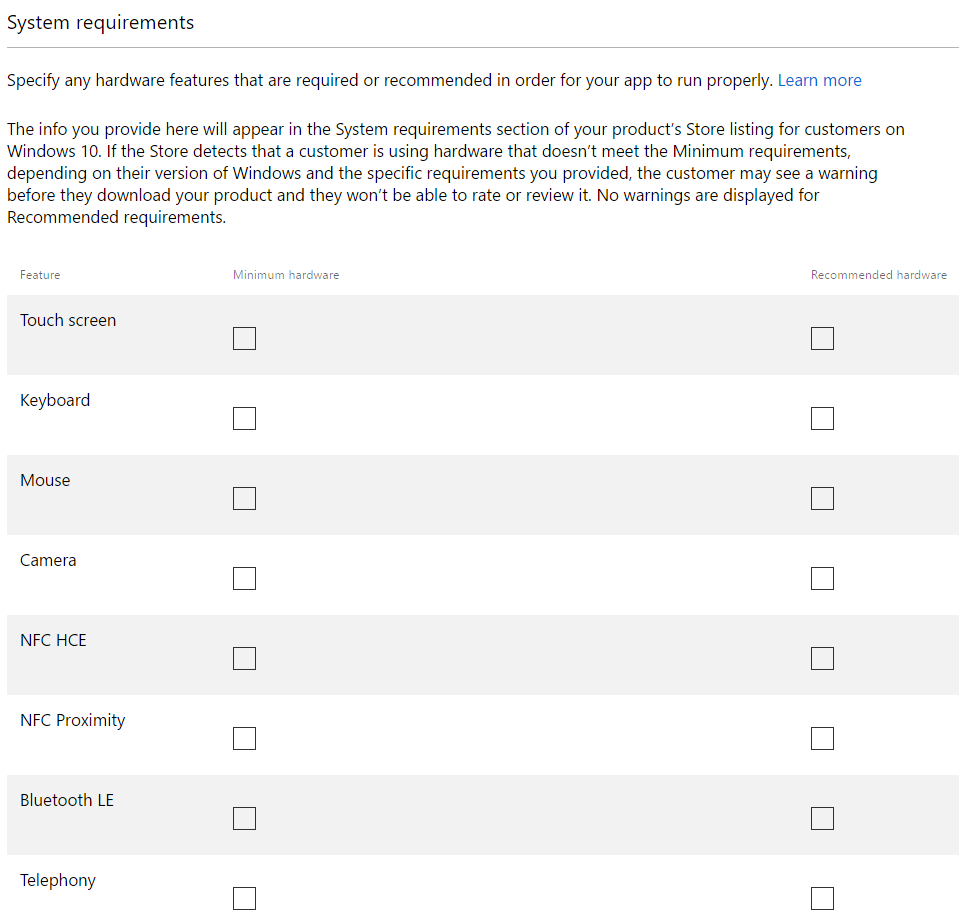The image depicts a vertical layout of a web page section, designed to assist developers in listing system requirements for their apps. The dimensions of the image suggest it is taller than it is wide, approximately 20-30% taller. The top left corner is marked with the title "System Requirements" in bold black text against a pristine white background. A horizontal line under the title signifies a new section below it.

In smaller black text, the introductory sentence directs developers to specify any hardware features required or recommended for optimal app performance. To the right of this sentence, the phrase "Learn more" is highlighted in blue, indicating a clickable link for additional information.

Beneath this, another paragraph elaborates that the details provided will appear in the system requirements section of the product store listing specific to Windows 10. It explains that if the store detects a customer's hardware does not meet the minimum requirements, a warning may appear before they can download the product, and they will be prevented from rating or reviewing the app. Contrarily, no warnings will be displayed for non-critical, recommended requirements.

Further down, the image contains a chart, neatly organized into three columns titled "Feature," "Minimum Hardware," and "Recommended Hardware," all written in small text. The chart alternates in background color between light gray and white rows, ensuring clarity and readability. The listed hardware components begin with a gray background for "Touchscreen," followed by "Keyboard," "Mouse," "Camera," "HFCHC," "NFC proximity," "Bluetooth LE," and "Telephony," each occupying a row and indicating specific hardware features.

This structured layout provides a clear, comprehensive guide for developers, ensuring their apps are appropriately matched with compatible hardware.